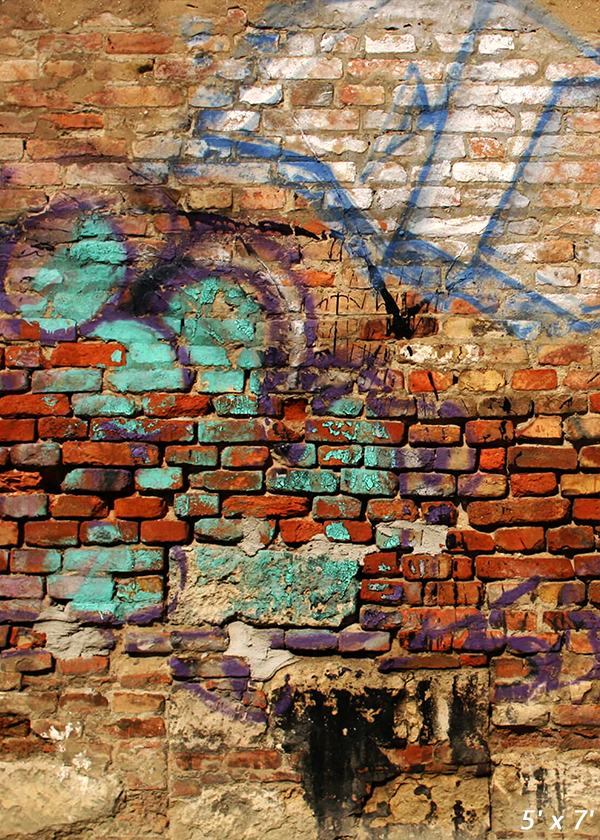The photograph is a detailed portrait of a graffiti-covered brick wall, likely an old building, adorned with various shades and tones of paint. The wall features three distinct sections: the lower part comprises loosely arranged, black-painted bricks interspersed with chunks of mortar and patches of graffiti; the middle part consists of uneven, dark red bricks marked with splotches of green and purple paint; and the top part showcases lighter, sandy-colored bricks embellished with blue, white, and purple graffiti that forms random lines and geometric shapes, although the specific designs remain indecipherable. The entire image is imbued with a sense of age and decay, as some areas of graffiti appear worn or scrubbed off. In the bottom right corner, digital text reads "5'x7'", possibly indicating the dimensions of the artwork or postcard print, adding to the intriguing, layered texture of the scene.